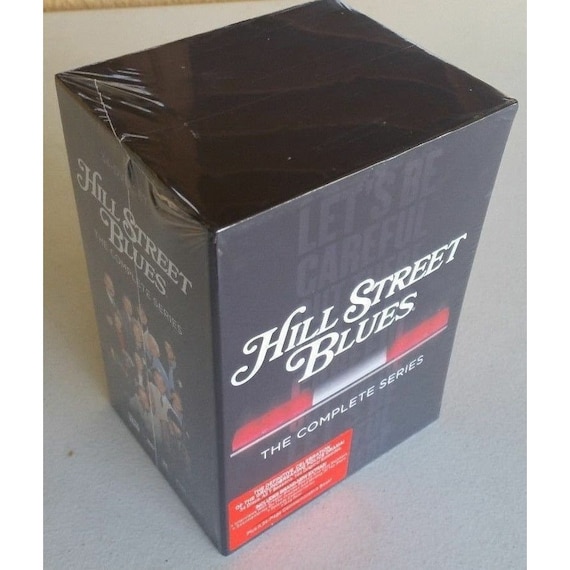This top-down photograph depicts a shrink-wrapped DVD box set of "Hill Street Blues: The Complete Series" resting on a white table. The box is positioned upright, revealing parts of two sides. The side facing the camera prominently displays the series title and a police car's lights image, with the phrase "let's be careful" faintly visible in the background in grayscale. A red sticker with white text is on the bottom left of the box, likely listing contents and features, though it's unreadable. The slightly visible left side repeats the series title and includes a photograph of the show's cast. This sealed DVD set, showcased on a gray table, remains unopened and pristine.